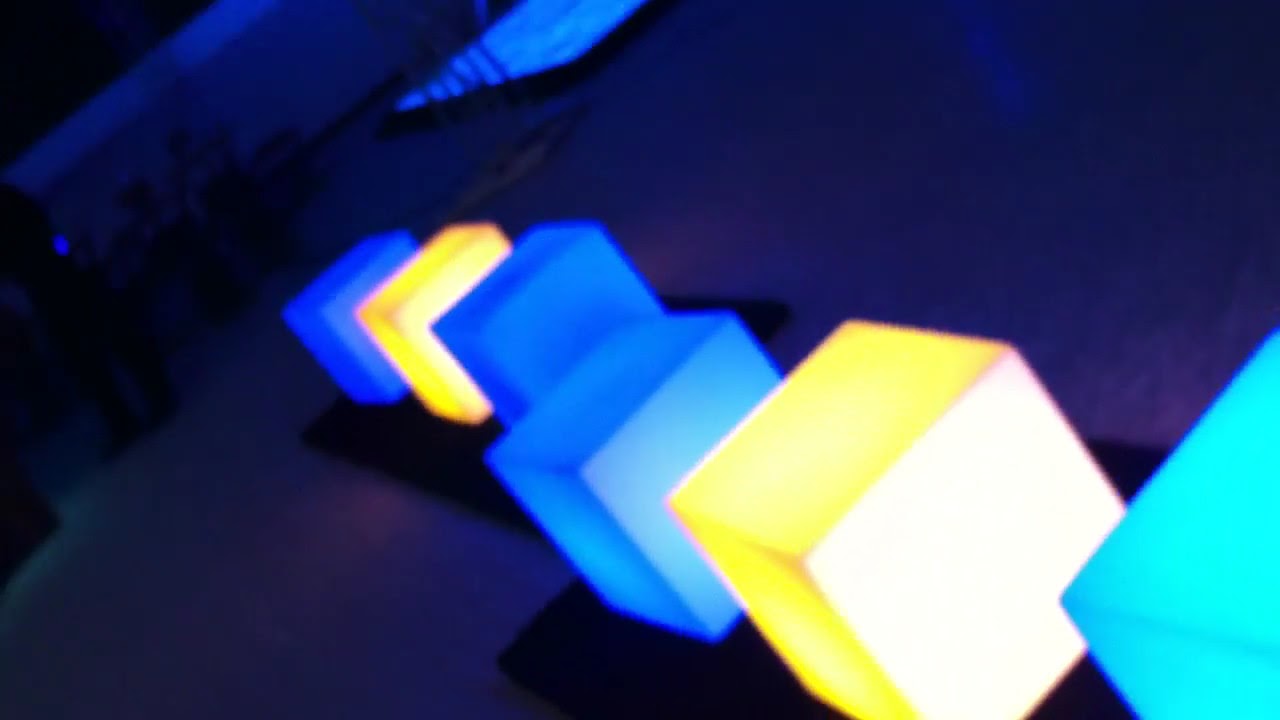In a dark, likely outdoor setting, the image captures a series of glowing cubes that appear to be lit from within, creating a striking pattern across the scene. The cubes are of varying colors, including one light blue, three regular blue, and two yellow. Positioned in an engaging composition, the cubes seem to form groups, possibly placed on black rectangular stands or surfaces, adding to the structured arrangement. Starting from the lower right-hand corner, one can see a light blue cube, followed by a yellow one with a nearly white face, and additional blue cubes. The entire scene seems to be viewed at a Dutch angle, with the cubes appearing to progress diagonally from the lower left towards the upper right. 

In the upper portion of the image towards the left, there is what looks like a lit-up blue pool, its water illuminated from beneath. The surrounding environment is subtly detailed with some inferred elements like plants and the outline of a wall in the upper left-hand corner, suggesting architectural features. The scene appears largely devoid of people, silhouetted perhaps by the dim lighting, enhancing the enigmatic and tranquil ambiance.